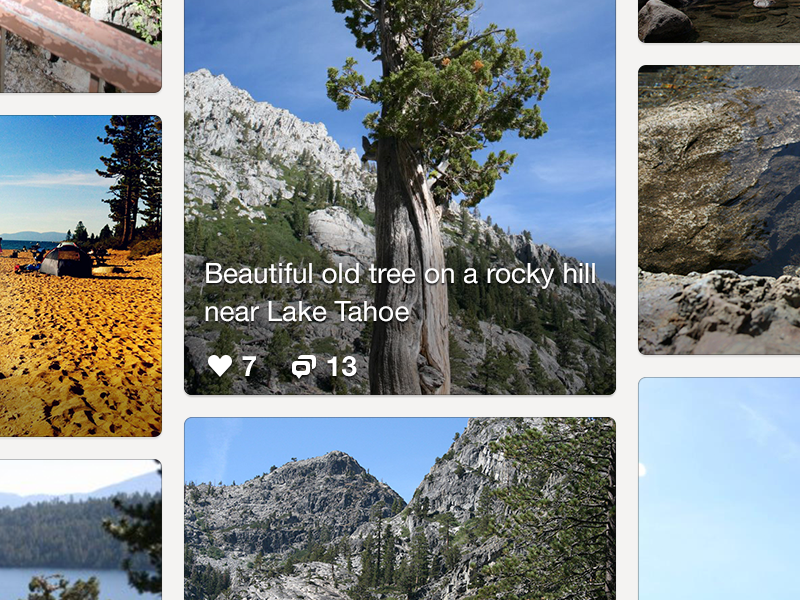A collage of eight photographs is arranged within the image. On the left side, there are three smaller photos, mirrored by three smaller photos on the right side, and in the center, there are one and a half larger photos stacked vertically. 

The top left photo appears to be of a pink-painted metal beam with trees or greenery in the background. Beneath it, the middle left photo depicts a sandy or yellow dirt landscape under a bright blue sky with scattered clouds and dark trees in the distance. The bottom left photo shows a snowy scene with mountains and dark trees.

In the center, the largest photo prominently features a caption reading, "Beautiful old tree on a rocky hill near Lake Tahoe." This striking tree is surrounded by seven heart icons and thirteen shared icons.

To the right of the large central photo, there is a smaller image at the top whose details are indistinct, but it possibly contains a large rock and a gravelly background. Beneath this, the middle right photo displays broken-up gravel with gold specks and corrosion. The bottom right photo showcases a serene view of blue skies with some white overcast clouds.

Finally, at the bottom center, another larger photograph captures a panorama of rocky mountains framed by lush tree landscapes. This detailed collage encapsulates diverse natural elements ranging from dense greenery and tranquil lakes to rugged mountains and expansive skies.